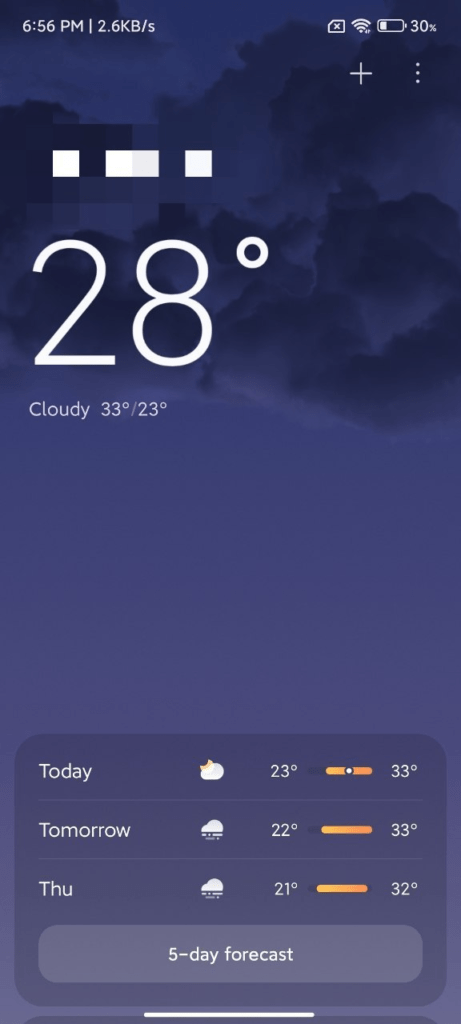The image displays a cell phone screen with a detailed weather forecast and various status indicators. In the upper left corner, the time is shown as 6:56 p.m. The right corner indicates a data speed of 2.6 KB/s, next to a square icon with an 'X', a Wi-Fi signal icon, and a battery level at 30%. Below this status bar, to the right, there is a plus sign and an ellipsis (three vertical dots). 

The weather section appears to be a widget with a partially white-out area below on the left, possibly an obscured widget or notification. It indicates the current temperature as 28 degrees and cloudy, with a high of 33 degrees and a low of 23 degrees, represented with a crescent moon icon.

The forecast for the upcoming days is detailed below:
- **Today**: Partly cloudy, 23 degrees, with temperatures ranging from a high of 33 degrees to a low of 20 degrees.
- **Tomorrow**: Cloudy, possibly rainy, 22 degrees with temperatures from 33 degrees to a low of 22 degrees.
- **Thursday**: Cloudy, possibly rainy, 21 degrees, with temperatures ranging from 32 degrees to a low of 21 degrees. 

At the bottom of the widget, there is a "Five-day forecast" button. The interface uses a combination of white, blue, blue-gray, orange, and yellow colors. The background features a night photograph with predominantly blue and gray clouds.